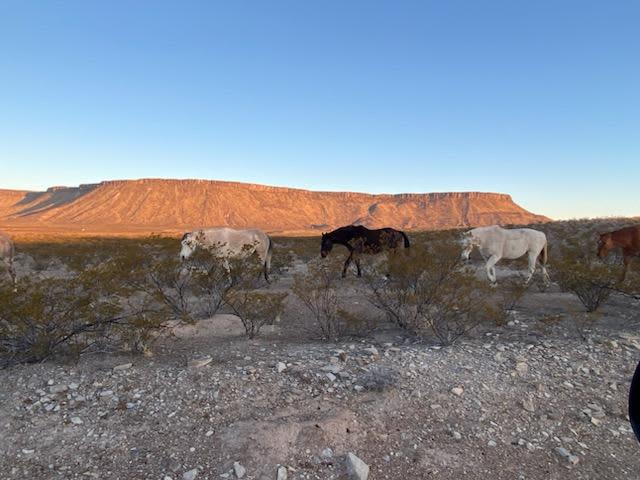In this image, captured outdoors in what appears to be the western or southwestern U.S., a striking landscape unfolds under a clear, blue sky devoid of clouds. The foreground reveals a gravel area composed of white and gray stones interspersed with spindly bushes featuring mostly black-brown branches and sparse green foliage. Beyond these bushes, a group of four wild horses walks in single file from right to left. The horses are arranged in this order: a white horse on the left, followed by a black horse, another white horse, and a partially visible brown horse. Beyond the horses, an expansive desert landscape stretches towards a distant, flat-topped mesa. The mesa, with its brown and tan hues, casts a prominent shadow on its left side while the right side is sunlit, suggesting the photograph was taken either shortly after sunrise or just before sunset, rendering a beautiful glow on the mountain.